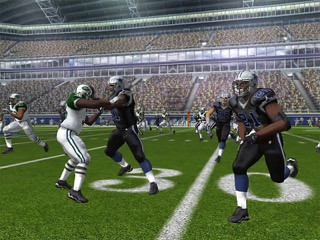This color screenshot is from a football-based video game, likely representing an NFL game. The image is a computer-generated scene depicting an intense moment on the 30-yard line in a brightly lit, packed stadium. In the foreground, multiple players from two different teams are engaged in the game, donning distinct uniforms: one team in white jerseys with black details, and the other in black jerseys with silvery accents. Notably, three primary players dominate the scene: two in black uniforms sprinting leftward, and one in a white uniform reaching out to stop them. Additional players wearing white uniforms are also visible, adding to the dynamic action. The stadium, filled with countless spectators, frames the dramatic action on the field, emphasized by the prominent "30" marker on the digital astroturf. The detailed, immersive graphics capture the intensity and atmosphere of a high-stakes football game.